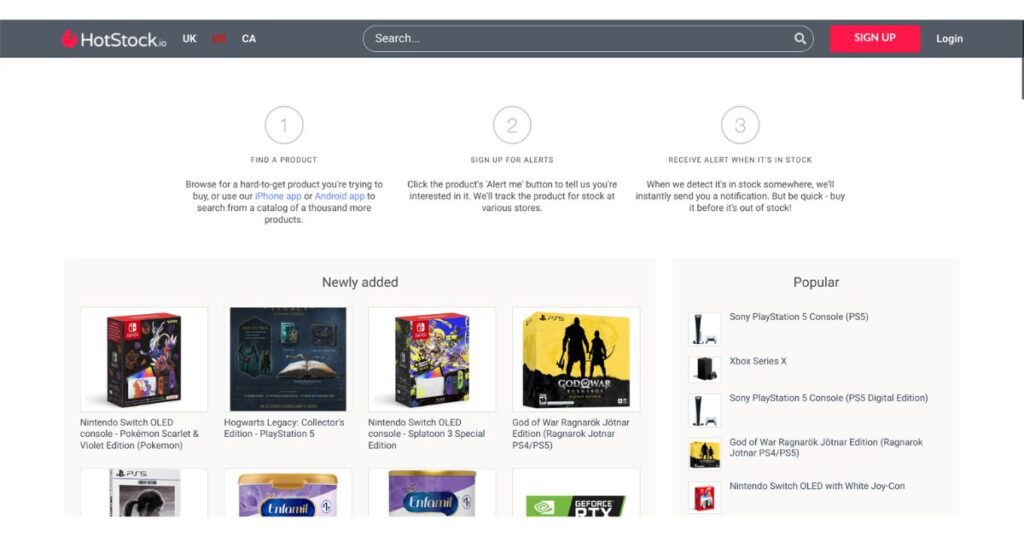The web page we're observing appears to feature a toolbar at the top, which includes the company name "Hot Stock" and offers a choice between UK and CA markets. Situated prominently is a search bar along with red buttons for signing up and logging in.

Scattered below the toolbar are new product listings, predominantly video games, showcasing titles such as a Nintendo Switch game, Hogwarts Legacy Collector's Edition for PlayStation, another Nintendo Switch game, and the God of War Ragnarök edition. Interestingly, the page also displays partially visible images of four additional games, suggesting a diverse range of newly added products.

Three circled numbers are prominently displayed, representing a streamlined process:
1. Find a Product: Users can browse for hard-to-get items or use the iPhone app.
2. Sign Up for Alerts: Stay informed by creating alerts for desired products.
3. Receive Alert When It's in Stock: Notifications are sent as soon as an item is available.

Further down the page, a "Popular" section lists high-demand items such as the Sony PlayStation 5 Console, Xbox Series X, and additional popular products including the Story PlayStation 5 console and God of War.

This detailed setup clearly caters to enthusiastic shoppers seeking exclusive or hard-to-find products.